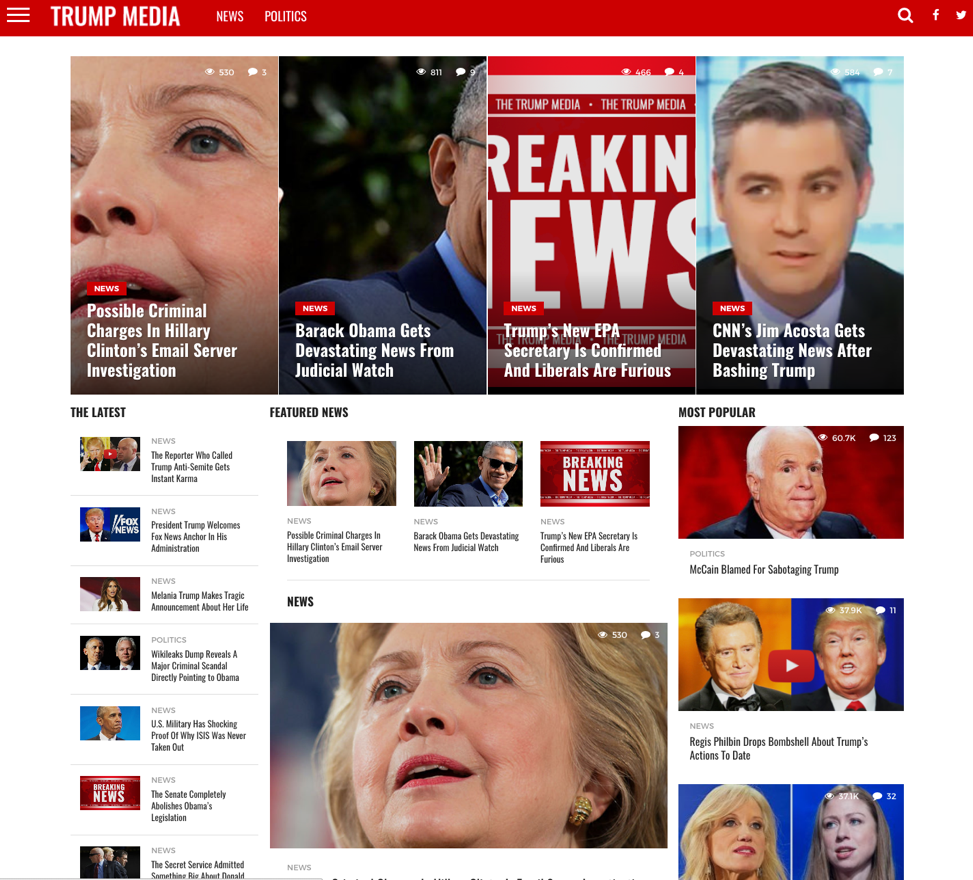This image is a detailed screenshot featuring various headlines often associated with sensationalism and partisan perspectives. 

In the upper left corner, the screen is branded with "Trump Media" on a red background, accompanied by the section title "News and Politics," suggesting a focus on political news pertaining to Donald Trump. This section appears to be a hub for aggregated stories centered on Trump and his political influence.

Key headlines include:
- "Possible Criminal Charges in Hillary Clinton's Email Server Investigation" suggesting legal troubles for Clinton.
- "Barack Obama Gets Devastating News from Judicial Watch," hinting at significant negative developments related to the former president.
- "Trump's New EPA Secretary is Confirmed and Liberals are Furious," indicating recent confirmation news and partisan reactions.
- "CNN's Jim Acosta Gets Devastating News After Bashing Trump," likely depicting a controversial figure within the media landscape.

On the right side of the screenshot:
- A prominent image of Senator John McCain is accompanied by a headline, "McCain Blamed for Sabotaging Trump," framed as a claim made solely by Trump.
- "Regis Philbin Drops Bombshell About Trump's Actions to Date" suggests a revelation from the TV host.
- In the bottom right corner, there's an image of Chelsea Clinton.

Other headlines on the left side include:
- "The Reporter Who Called Trump Anti-Semite Gets Instant Karma."
- "President Trump Welcomes Fox News Anchor in His Administration."
- "Melania Trump Makes Tragic Announcement About Her Life."
- "WikiLeaks Dump Reveals a Major Criminal Scandal Directly Pointing to Obama."
- "U.S. Military Has Shocking Proof of Why ISIS Was Never Taken Out."

These headlines are typical examples of the sensationalist and frequently disputed content found on certain partisan news platforms, often criticized as "fake news" and seen as misleading or unverified.